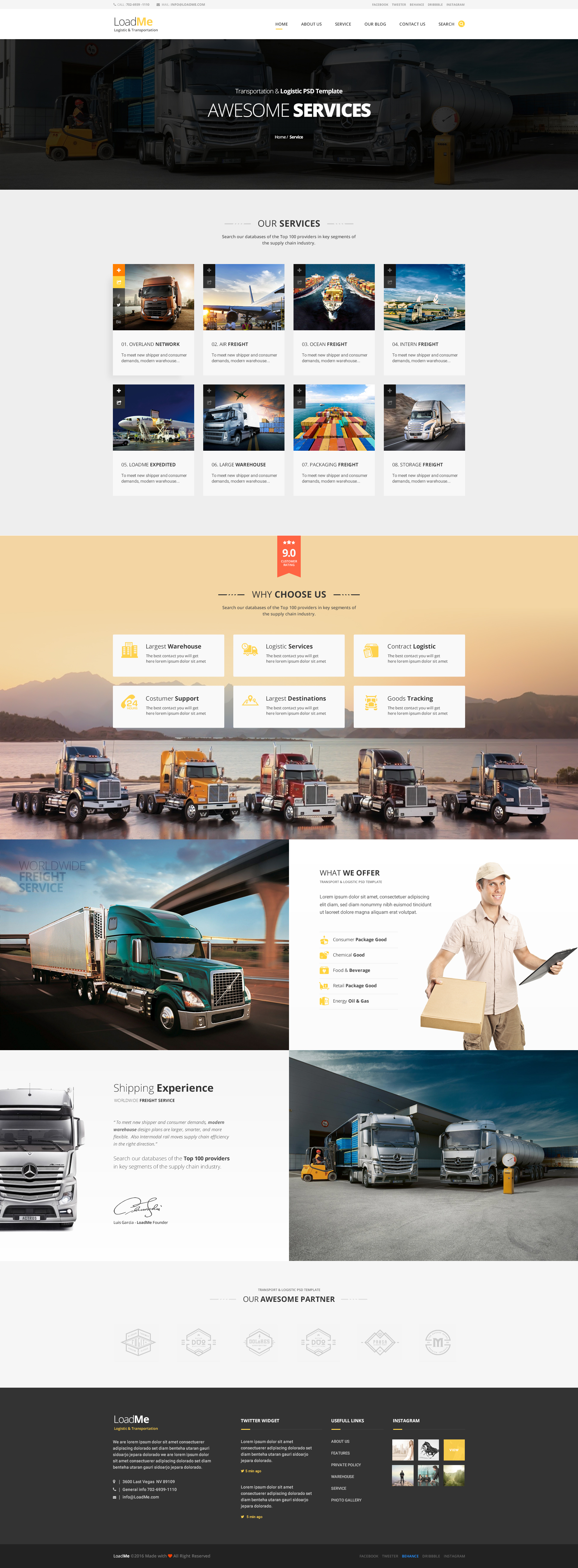A screenshot of the LoadMe website, dedicated to shipping and logistics services. The navigation bar at the top includes links to 'Search,' 'Contact Us,' 'Our Blog,' 'Service,' 'About Us,' and 'Home.' The main section highlights their transportation and logistic PSD template titled "Awesome Services." The services listed include Overland Network, Air Freight, Ocean Freight, Internal Freight, LoadMe Expedited, Large Warehouse, Packaging Freight, and Storage Freight. The site features various images of ships, planes, semi-trucks, cargo ships, and other shipping methods. Detailed information is provided on their offerings, which encompass consumer packaged goods, chemical goods, food and beverages, retail packaged goods, energy, oil, and gas. Additionally, the website emphasizes their worldwide freight service and extensive shipping experience. At the bottom of the page, contact information is available, indicating that the company is based in Las Vegas.